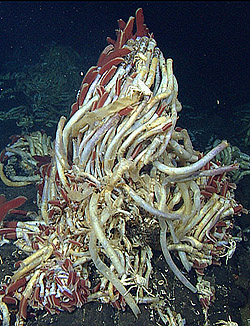This is a highly detailed, portrait-oriented color photograph depicting an underwater volcanic vent community. At the center of the image, a conical formation of brightly colored, thin, ribbon-like worms—predominantly silver, gold, and red—intertwine and cluster together, creating the appearance of a writhing, tangled mound. These worms look almost snake-like, contributing to a chaotic yet mesmerizing scene. Surrounding the base of this formation are cream-colored, crab-like creatures with long, segmented legs, adding to the complexity of the underwater ecosystem. The background is black, likely indicating the depths of the ocean, with additional, less focused objects that hint at the vastness and diversity of life on the seafloor. The photographic style is one of realism, capturing the intricate details of this fascinating deep-sea environment.